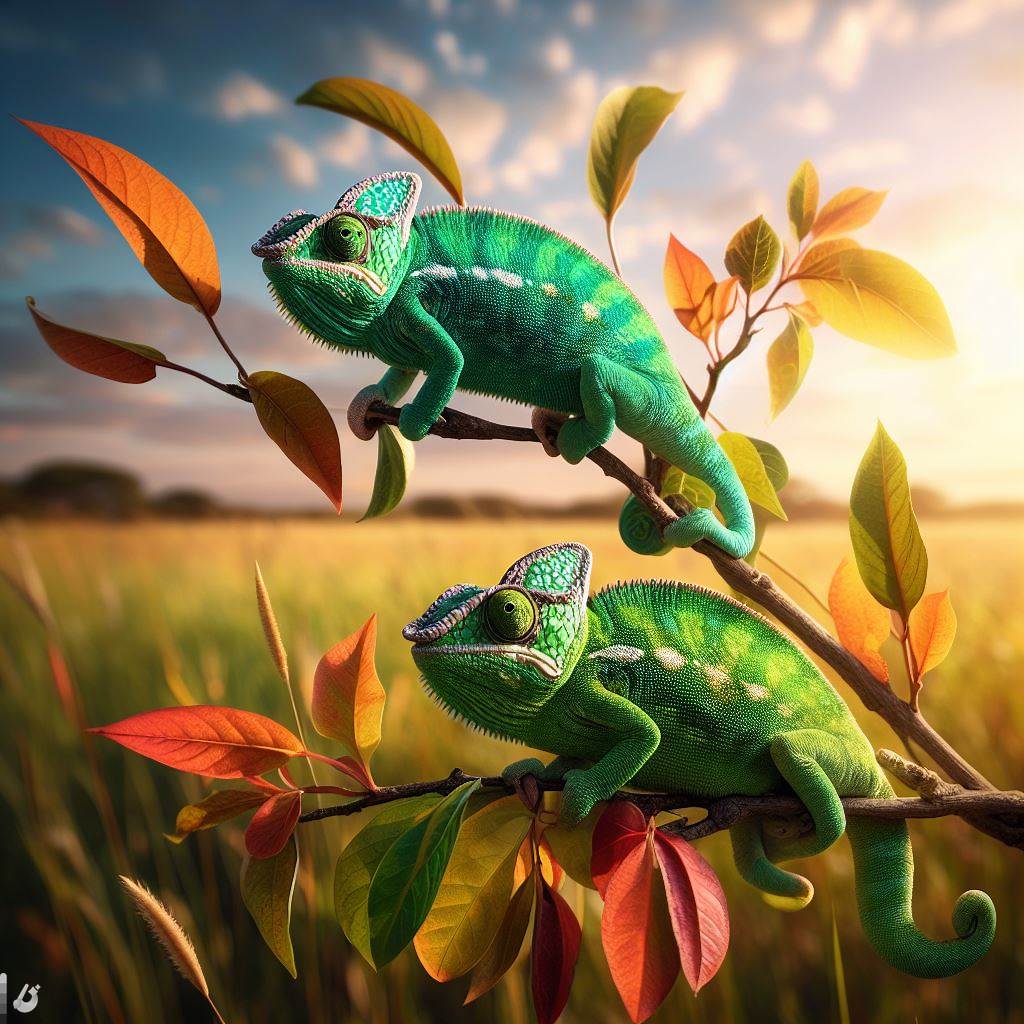This highly detailed digital artwork, likely AI-generated due to certain inconsistencies, depicts two lizards perched on a forked branch adorned with leaves in varying shades of green, yellow, and orange. The lizards, whose exact species might be chameleons or iguanas, are gripping separate sections of the branch—one positioned slightly above the other. Both lizards have a green hue, with one showing more blue undertones, and display cartoonish features, including large eyes and intricate facial decorations. The backdrop features an out-of-focus prairie landscape with a thin band of mountains or forested areas halfway up the image, transitioning into a blue sky filled with clouds. A solar flare on the right side of the image suggests either sunrise or sunset, illuminating the scene with a warm, sunny glow.